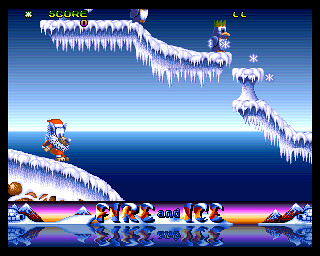The image captures a moment of gameplay set in a wintery, whimsical landscape. At the top of the screen, the word "Score" is displayed in green text. Below that, a series of ledges resembling icicles in shades of white and blue extends downwards. Perched on one of these ledges is an owl-like figure, adorned in blue with an orange beak and a crown that appears to be tinged with green. A distinctive snowflake mark decorates its body. Adjacent to the owl on the same ledge is another character, featuring a navy appearance and a white beard, adding to the icy theme.

Further down is another icicle ledge, also white and blue, sprinkled with snowflakes. Positioned below this ledge is a friendly-looking, furry monster character. This creature, with its white and blue fur and large googly eyes, is dressed festively in a Santa outfit, complete with a red and white hat and matching attire. It stands on an ice ledge, behind which a serene blue water body is visible.

Towards the bottom of the image, vibrant graphics spell out "Fire and Ice" in a blend of blue, white, and orange hues. The background behind the text is a striking mix of purples and oranges. This backdrop features elements of an arctic scene, including igloos and snow-covered mountains. The setting is beautifully reflected in an adjacent body of water, echoing the orange and purple tones of the sky.